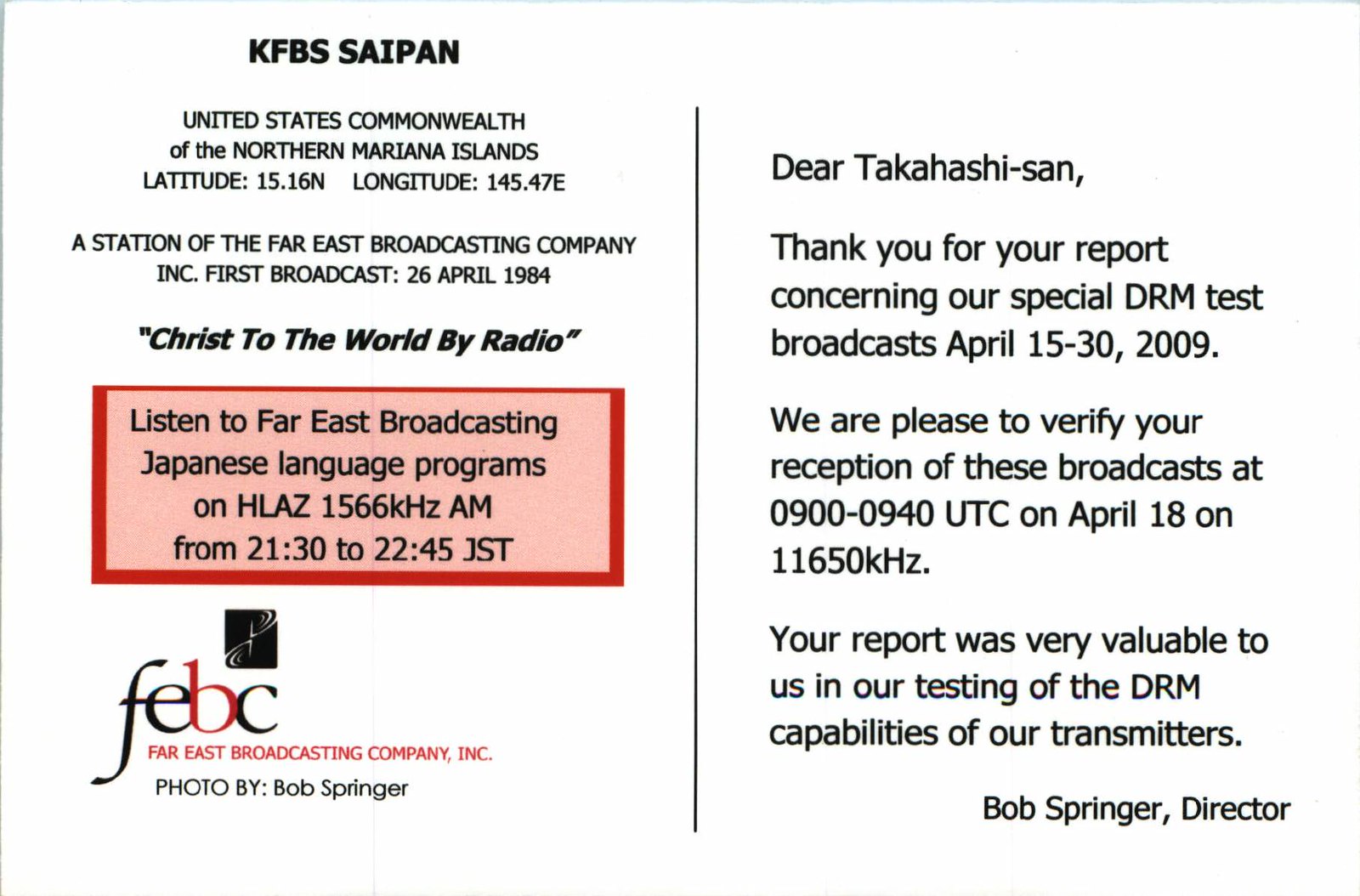The image is one side of a postcard divided by a vertical black line down the middle. On the left side, the text reads: "KFBS Saipan, United States Commonwealth of the Northern Mariana Islands. Latitude 15.16 and Longitude 145.47. A station of the Far East Broadcasting Company, Inc. First broadcast 26 April 1984. Christ to the World by Radio." Below this, a rectangular box with a light pink fill and red border contains the text: "Listen to Far East Broadcasting Japanese Language Program on HLAZ 1566 KHz AM from 2130 to 2245 JST." Under the box is a logo of the company, followed by the inscription: "FEBC, Far East Broadcasting Company, Inc. Photo by Bob Springer."

On the right side of the vertical line, the text is: "Dear Takahashi-san, thank you for your report concerning our special DRM test broadcast April 15-30, 2009. We are pleased to verify your reception of these broadcasts at 0900-0940 UTC on April 18 on 11650 KHz. Your report was very valuable to us in our testing of the DRM capabilities of our transmitters. Bob Springer, Director."